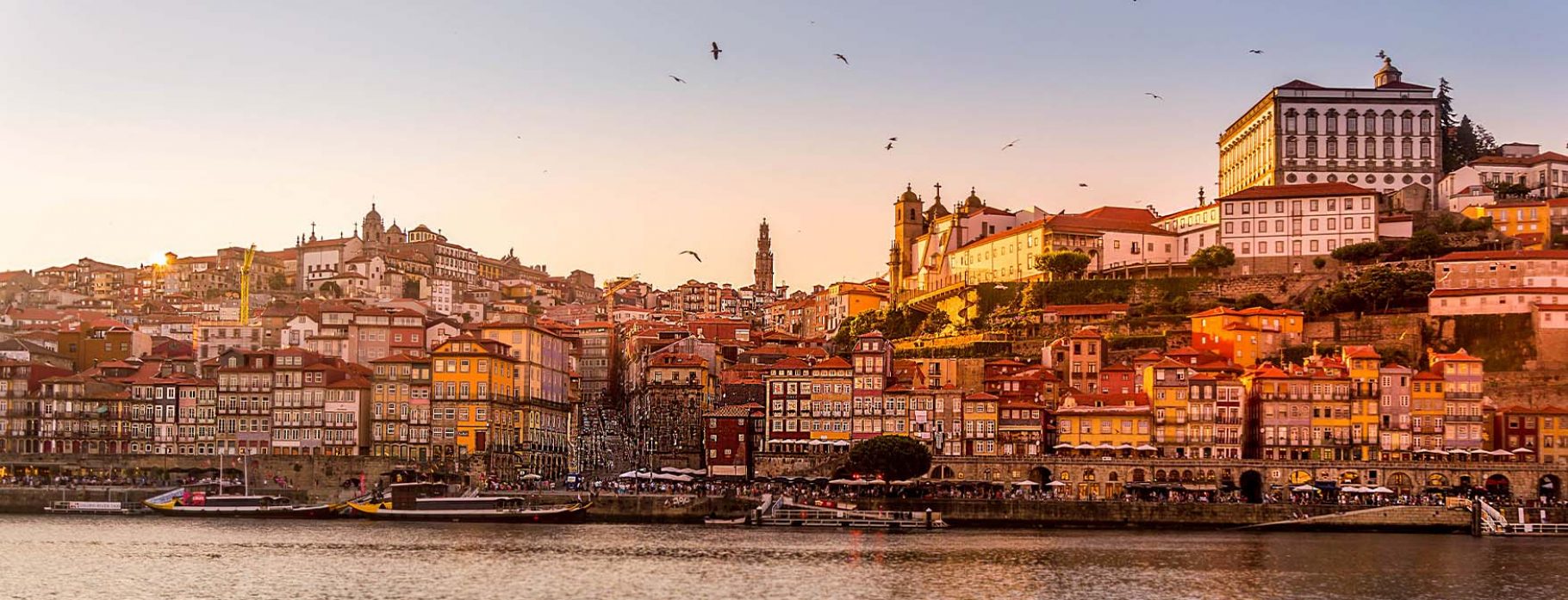This stunning photograph captures a bustling European port city, likely Italian, built upon a series of hills that rise from the waterfront. The scene is bathed in the warm glow of the golden hour, with the sun setting on the left horizon, casting a spectrum of colors from light white to dark blue in the sky. The calm water, possibly a seaport but open to being a lake or river, gently reflects the light, with small ripples and scattered birds enhancing the serene atmosphere.

The lower part of the image showcases a bustling dock filled with various boats, some of significant length, hinting at their cargo or fishing purposes. The harbor is lined with a multitude of narrow buildings, closely packed together, their aged facades adding a historical charm to the scene. Ascending the hills, the cityscape is dense with structures, including several large buildings that rise five to six stories high.

Dominating the skyline are notable landmarks like church steeples, specifically a prominent church tower at the center and another church with a visible cross on its feature to the right. Towards the far right of the photo stands a distinguished white building with windows, set against the backdrop of a darker blue section of sky. This composition, teeming with architectural variety and life, conveys a rich, cultural tapestry indicative of a thriving, populated port city.